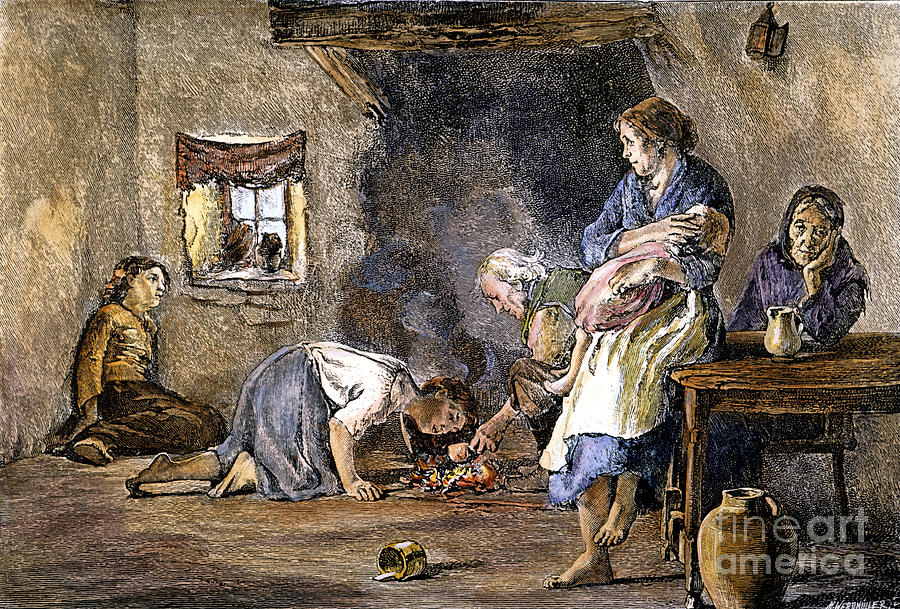The image appears to be a detailed scan of a painting depicting a sparse room with minimal furnishings, including a table and a chair. On the left side of the room, a young girl sits on the floor in a corner, seemingly lost in thought. Next to her, another girl is kneeling and appears to be picking something up from the ground. Beside her, a man is also squatting, occupied with picking up what looks like a small container or cup. On the right side, a woman is leaning against the table, cradling a baby in her arms. Seated on a chair, an elderly woman rests her arm on the table. The table surface features a small container, with a larger one placed underneath. There are distinct details such as a small window, a door centrally positioned, a cat sitting on a ledge, and an inscription in the bottom right corner that reads "Fine Art America." Notably, the room's overall atmosphere is humble and intimate, evocative of an old painting's charm.